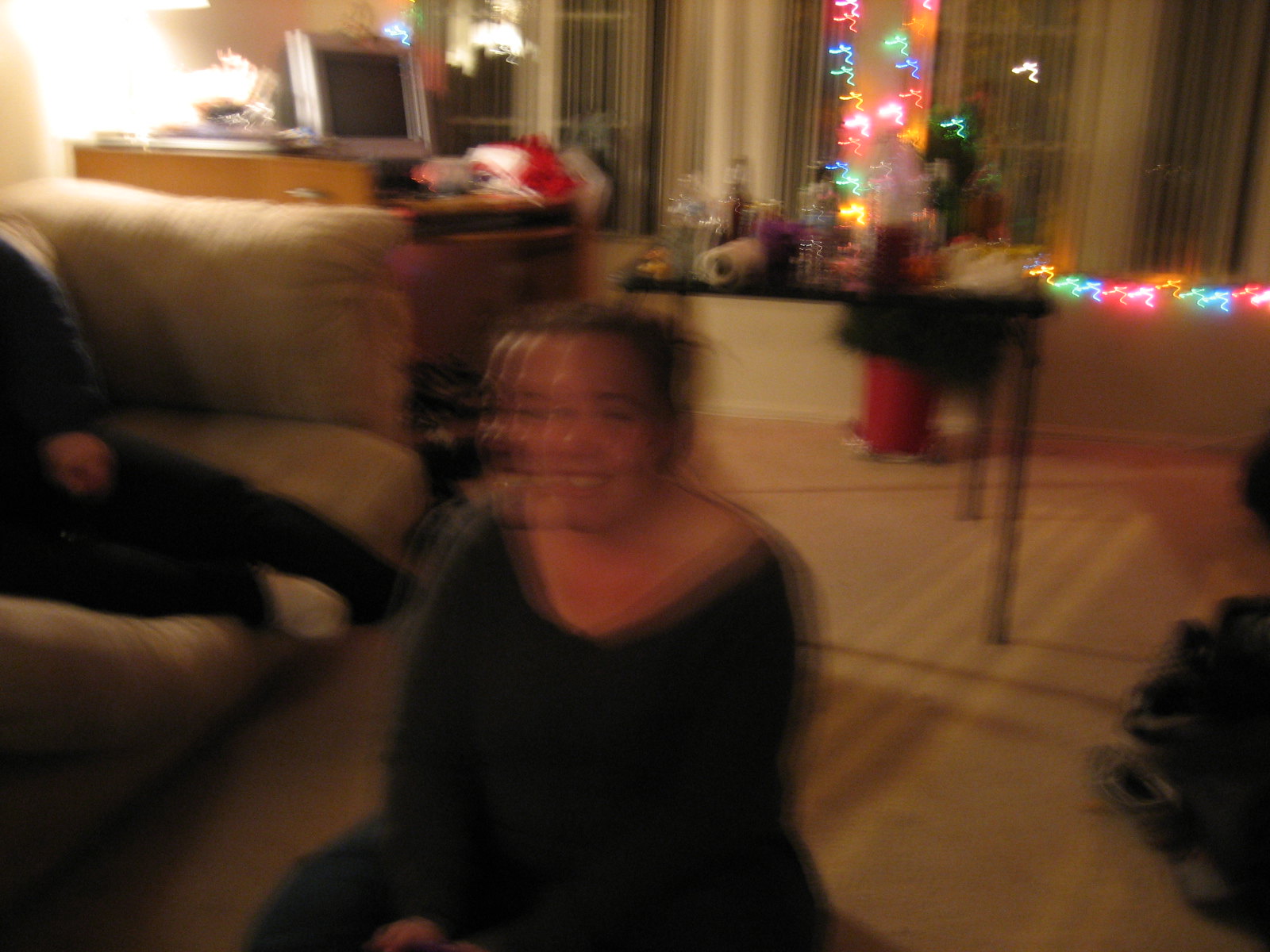In this festive, albeit slightly blurry, image, a woman with brown hair and a v-neck shirt sits amid a cozy holiday setting, potentially opening Christmas presents. She is wearing brown pants and a green sweater, and her cheerful demeanor complements the seasonal atmosphere. Behind her, a decorated Christmas tree adds to the festive spirit, positioned next to a wooden table. To her left, a male figure is comfortably seated on a couch. The room is warmly lit by red, rainbow-colored Christmas lights adorning Venetian-style blinds in the window. A nostalgically lit Santa Claus figurine stands on a wooden computer desk in the background, completing the charming Christmas scene.